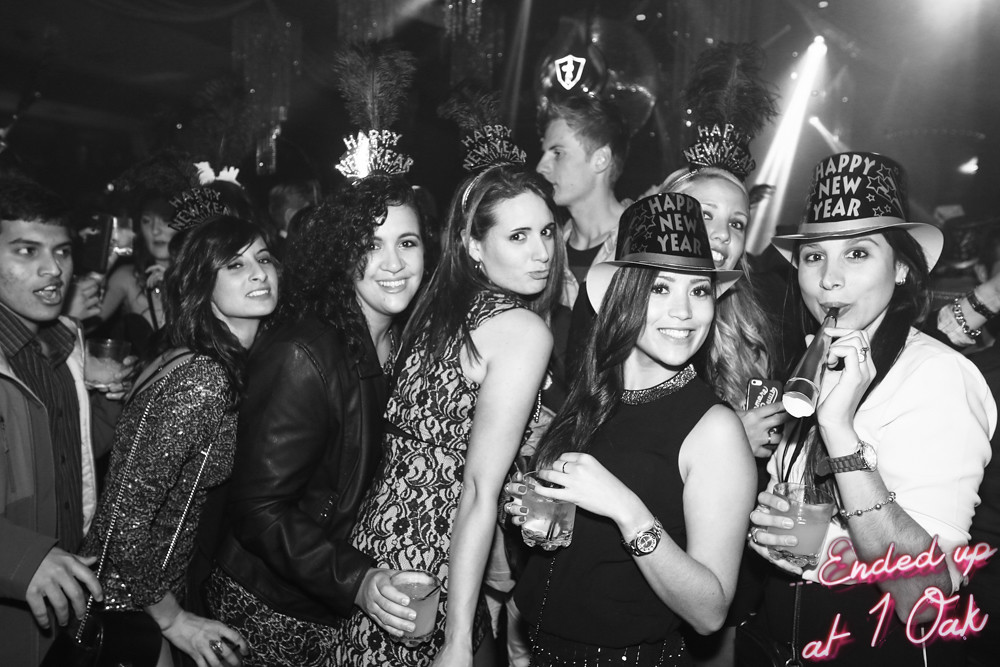This black-and-white photograph captures the lively essence of a New Year's Eve party, with a group of mid-20s partygoers tightly huddled together for the camera. The scene is likely on a dance floor, illuminated by spotlights visible from the ceiling or walls. At the forefront are five women, all donning "Happy New Year" party hats—some fashioned like tiaras. One girl has a party horn in her mouth, while another girl wearing a black leather jacket holds a drink. Among them, another woman also clutches her drink. A sixth woman is slightly behind the central group, and on the far left, a man appears to be inserting himself into the shot. Further back, another taller man looks away from the camera, adding depth to the background, which is filled with more party revelers and stage lights. Overlaying the lower right corner of the image is a neon pink text that reads, "ended up at one oak," lending a modern, stylish touch to this festive New Year's snapshot.